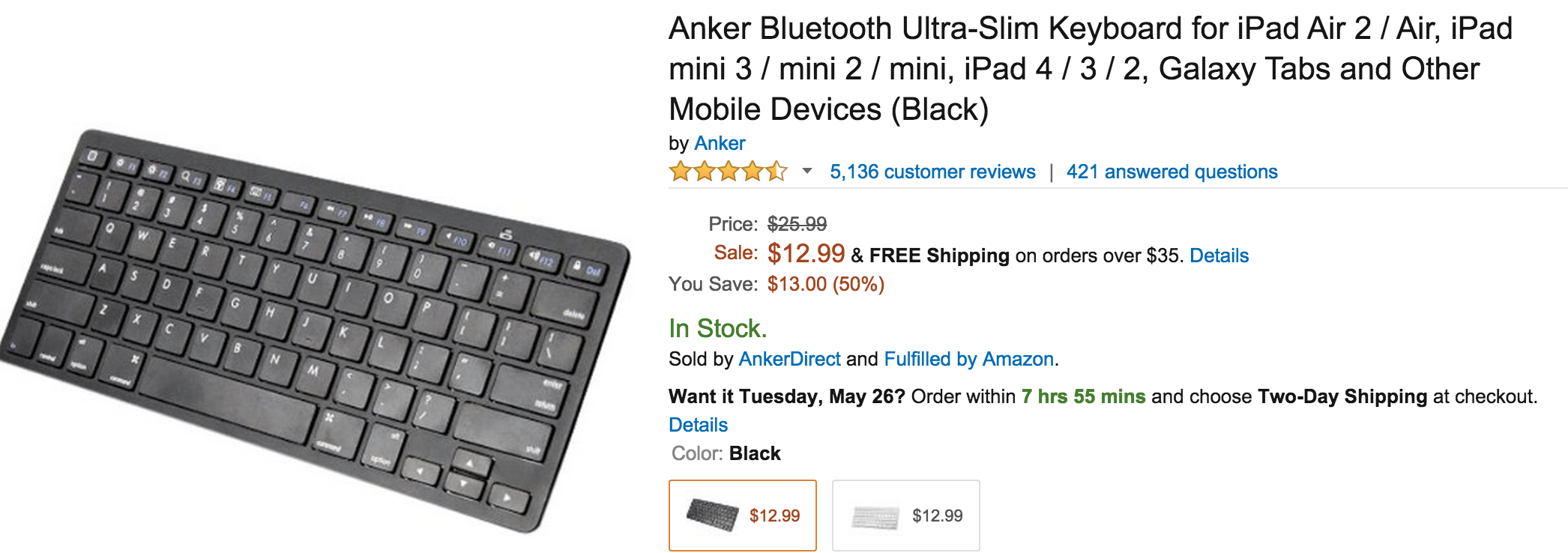Here is a detailed and cleaned-up caption based on the provided information:

---

This image is a detailed screenshot of a product page on Amazon for the Anker Bluetooth Ultra Slim Keyboard, designed for various iPad models, including the iPad Air 2, iPad Mini 3, Mini 2, Mini, iPad 4, 3, and 2, along with compatibility for Galaxy tablets and other mobile devices. The product featured is the black version, manufactured by Anker. It has received high customer satisfaction, boasting a rating of 4.5 out of 5 stars from 5,136 reviews and 421 answered questions.

The original price of this keyboard is listed as $26.99, but it is currently on sale for $12.99, a substantial 50% discount. The new, reduced price is highlighted in red, and the offer includes free shipping on orders over $35. The product is in stock and available for purchase from Anker Direct, with fulfillment by Amazon.

There are two color options available for this keyboard: black and white, both priced at $12.99. The product image displayed on the left shows the black keyboard featuring black keys with white letters and numbers for clear visibility.